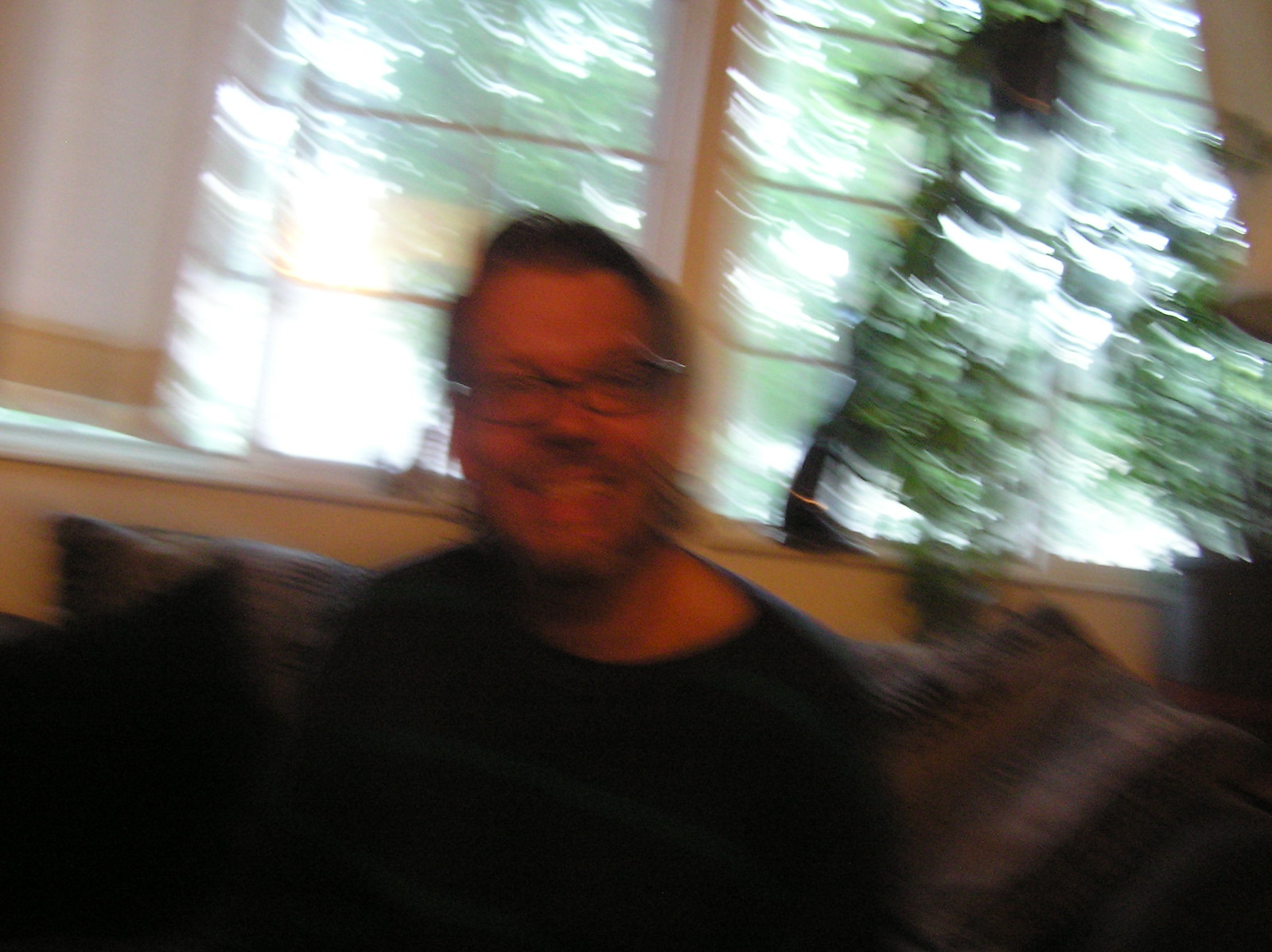In this slightly blurred and dimly lit photograph, a close-up captures a smiling man gazing directly at the camera. His somewhat long hair is slicked back at the forehead with some sort of hair product, accentuating his stylish appearance. He sports black-framed glasses that complement his well-tanned complexion, along with a neatly groomed beard and mustache. The man is dressed in a dark, navy blue pullover shirt adorned with light blue or grayish horizontal stripes, and the boat neck of the shirt adds a subtle touch of flair.

He is seated comfortably on a couch that is decorated with an array of throw pillows, including a prominent black one. The couch itself boasts an intricate purple and black patterned fabric. Behind him, a pale yellow wall blends into the background, punctuated by a large multi-paned window that streams in an abundance of natural light. Through the window, the lush greenery of several trees can be seen, adding a refreshing contrast to the cozy indoor setting.